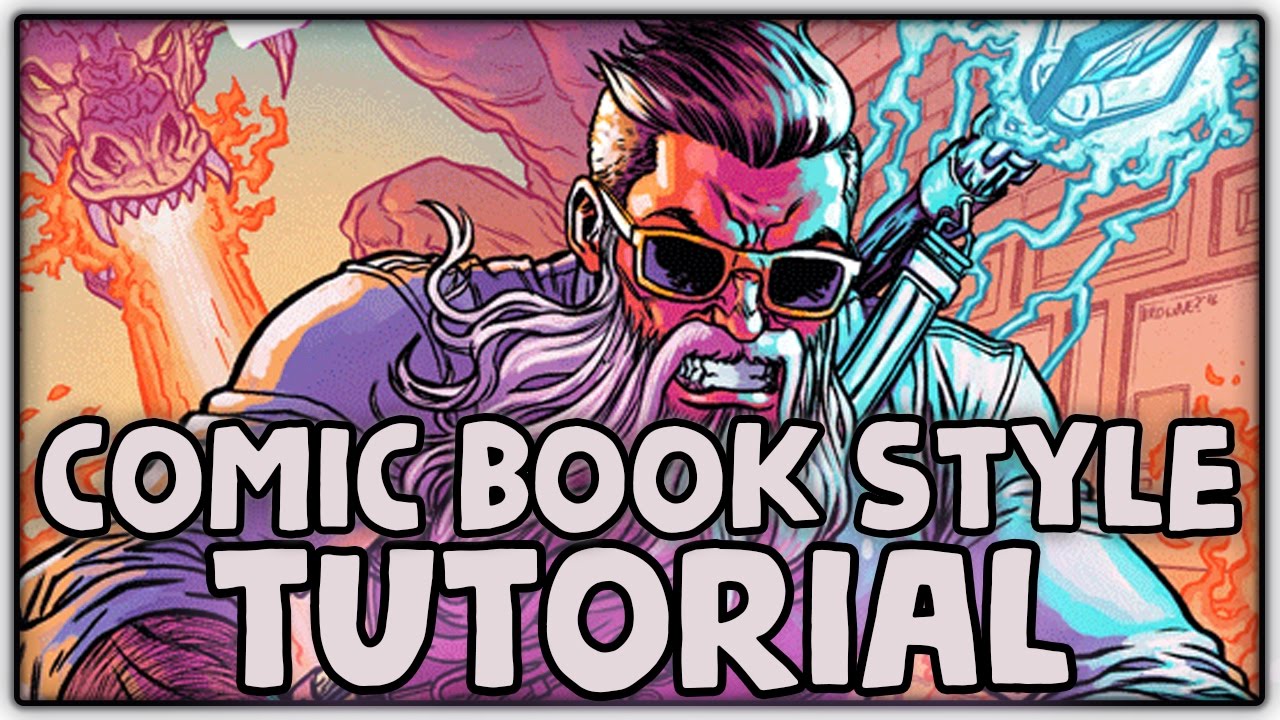In this vibrant comic book-style illustration featuring a tutorial text, we see a dynamic scene characterized by vivid colors such as orange, yellow, purple, pink, neon blue, beige, tan, and brown. The focal point is an intense confrontation between a bearded, sunglasses-wearing man wielding a gleaming, lightning-emitting staff, and a ferocious dragon whose head occupies the top left corner, unleashing a torrent of blazing fire. The man, positioned centrally and oriented downward, appears ready for battle atop what could be a motorcycle, suggested by his posture and surroundings. The rocky terrain and a storefront with doors and windows flank him on either side, adding context and depth. The bottom middle of the image is dominated by bold, white bubble letters bordered in black, spelling out "Comic Book Style Tutorial," anchoring the theme of the illustration.